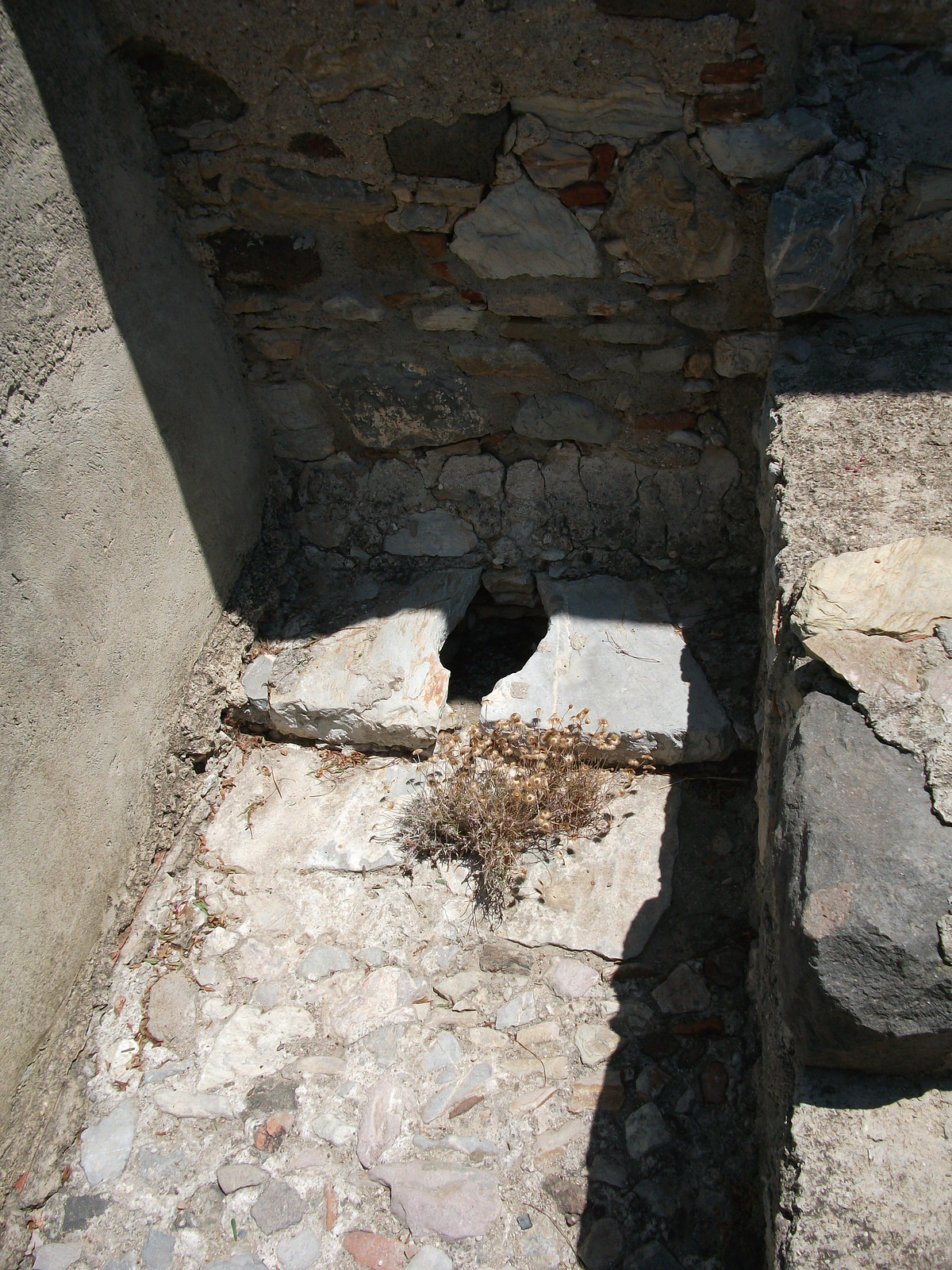This image captures a part of the interior of a rustic building constructed with rock and concrete, taken during the day as indicated by the sunlight casting shadows on the bottom of the rocks. The structure features prominently in the frame, with a concrete wall on the left-hand side. Adjacent to it, a wall comprises a mix of concrete, brick, and varying shades of rock, including lighter browns, whites, grayish blues, salmon, and a few red bricks, creating a textured and rustic appearance. The floor consists of large gray concrete slabs with slight gaps between them, transitioning into an assortment of different shapes of gray rock. On the right, there appears to be a half concrete wall. There is a pit-like formation going downwards at the center with a noticeable hole at the bottom, resembling a toilet pit, flanked by a dry-looking plant. The overall feel is an earthy blend of stone and concrete elements, enhanced by the diverse hues of the rocks and bricks.